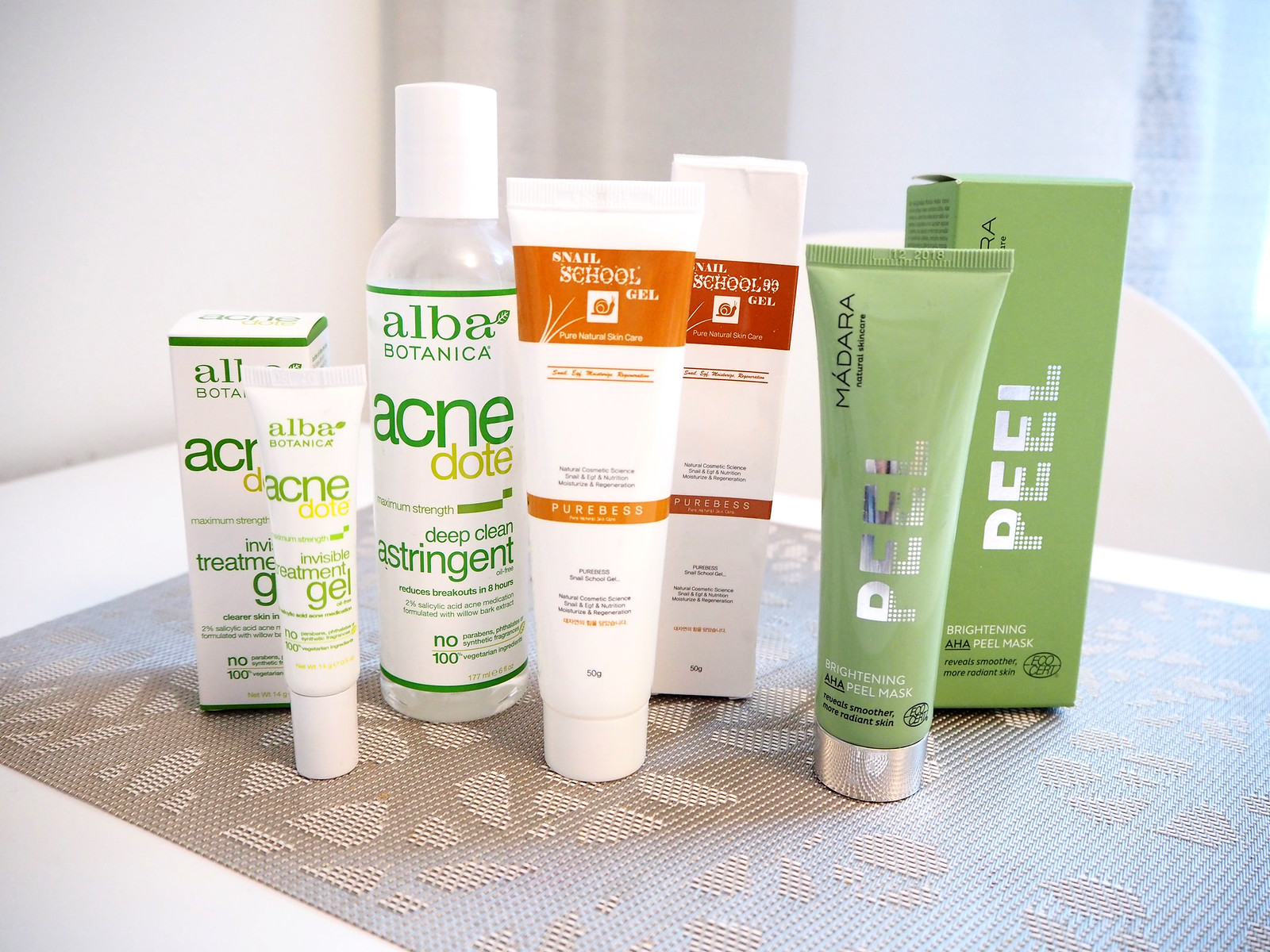This detailed close-up photograph features seven skincare products meticulously arranged on a silver mat with an abstract design, placed on a white surface. Shot from a slightly elevated angle, the composition includes three Alba Botanica products grouped together on the left. A white box labeled "Invasive Treatment Gel" in kelly green lowercase font is situated at the back, with a matching green-labeled tube of "Acne Dote" standing on its cap in front of it. Adjacent is a tall, clear plastic bottle with a screw cap, also from Alba Botanica, labeled "Acne Dote Deep Clean Astringent."

Central to the arrangement is a product in a white tube with sienna orange accents and a logo of a snail, labeled "Snail School Gel." Its corresponding white box, featuring the same design and deeper orange banding, is positioned to its right.

Completing the group on the right is a medium green tube of another skincare product labeled "Peel" in shiny silver letters. This tube, topped with a silver cap, stands in front of its matching green box, which bears the same "Peel" font and the brand name "Madara."

In the background, a window is visible to the right, flanked by white walls. Sitting before the window is a hemispheric white plastic object, adding an additional layer of visual interest to the composition.